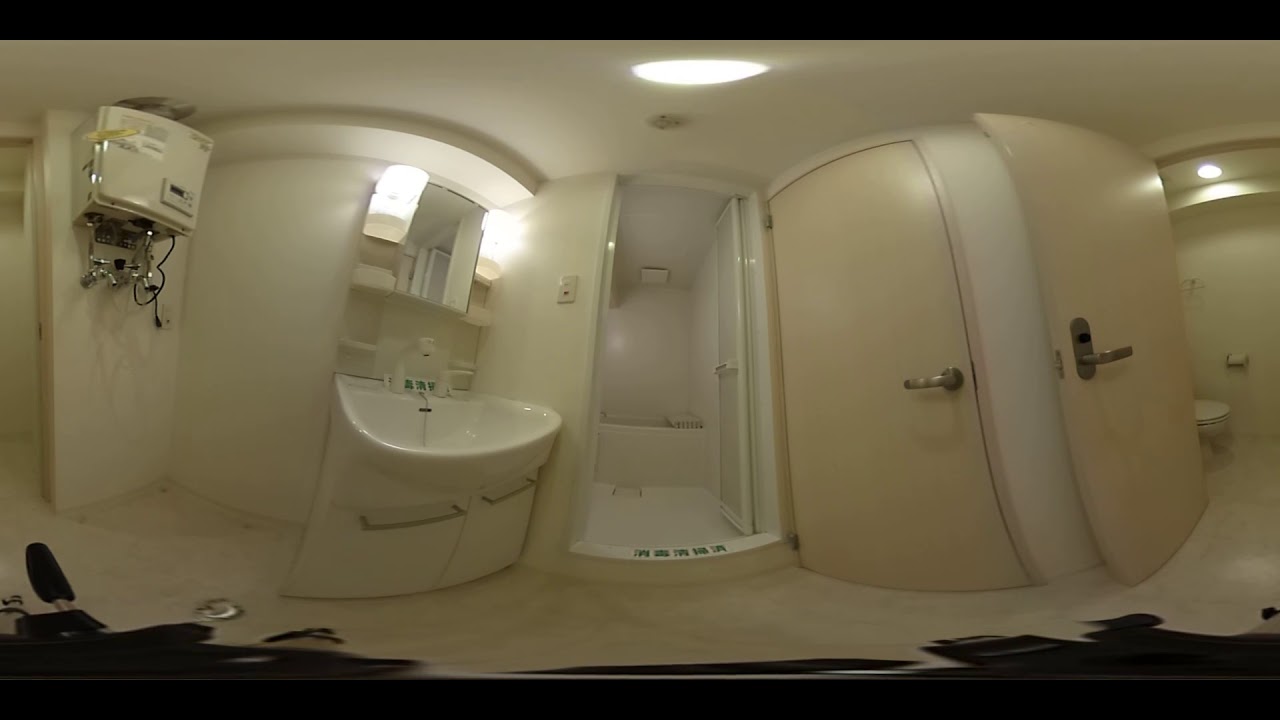The image captures a detailed 360-degree view of a clean and well-lit bathroom with cream-colored walls and surfaces. On the right side, there's an open door revealing a toilet and a wall-mounted toilet paper holder. Adjacent to this is a closed door of a similar color. Central to the image, you see what appears to be a standing shower or a shower cabin. To the left of the shower is a large, white bathroom sink, above which hangs a mirror flanked by two bright lights. Continuing left, there's a square-shaped, wall-mounted machine, possibly a water heater, though it appears unplugged with visible pipes. The entire bathroom is spacious, with ample lighting and a tidy appearance.